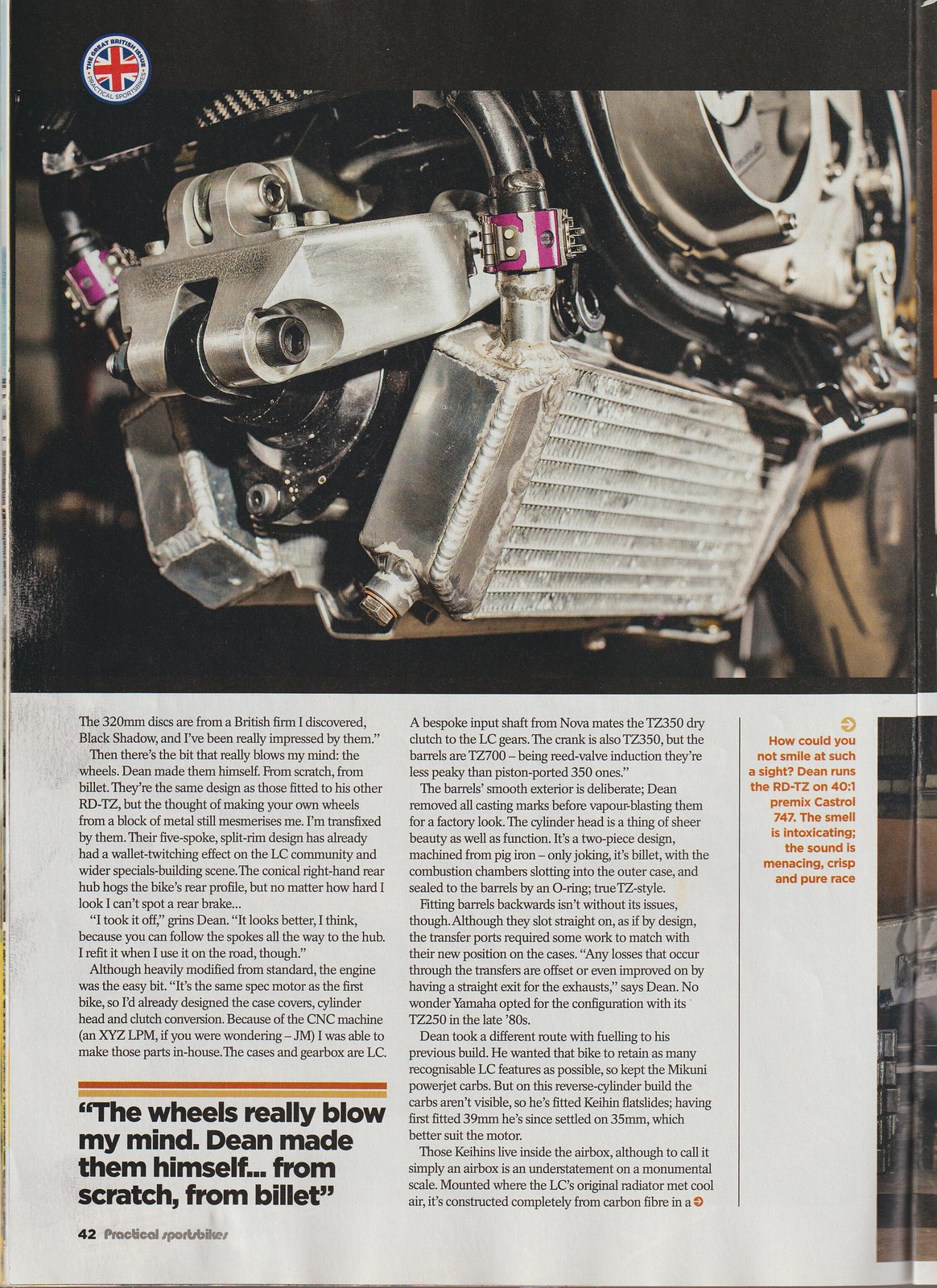The image depicts a detailed photograph of a car or motorcycle engine, featured on page 42 of Practical Sports Bikes magazine. The engine itself is predominantly silver and black, with notable magenta clamps holding its components together. Positioned horizontally at the top half of the page, the engine is intricately detailed, showcasing nuts, bolts, filters, and what appears to be a carburetor. In the top left corner, there is a circular logo of the British flag, labeled "The Great British Issue." Accompanying the image is an article filled with text on a white background adorned with red and yellow lines. Highlighted quotes emphasize the craftsmanship and impact of the machine, stating, "The wheels really blow my mind. Dean made them himself from scratch, from billet," and, "How could you not smile at such a sight? Dean runs the RD-TZ on 40 to 1 premix Castrol 747. The smell is intoxicating, the sound is menacing, crisp and pure race." This visually striking and informative layout captures the essence of high-performance engineering and British automotive pride.